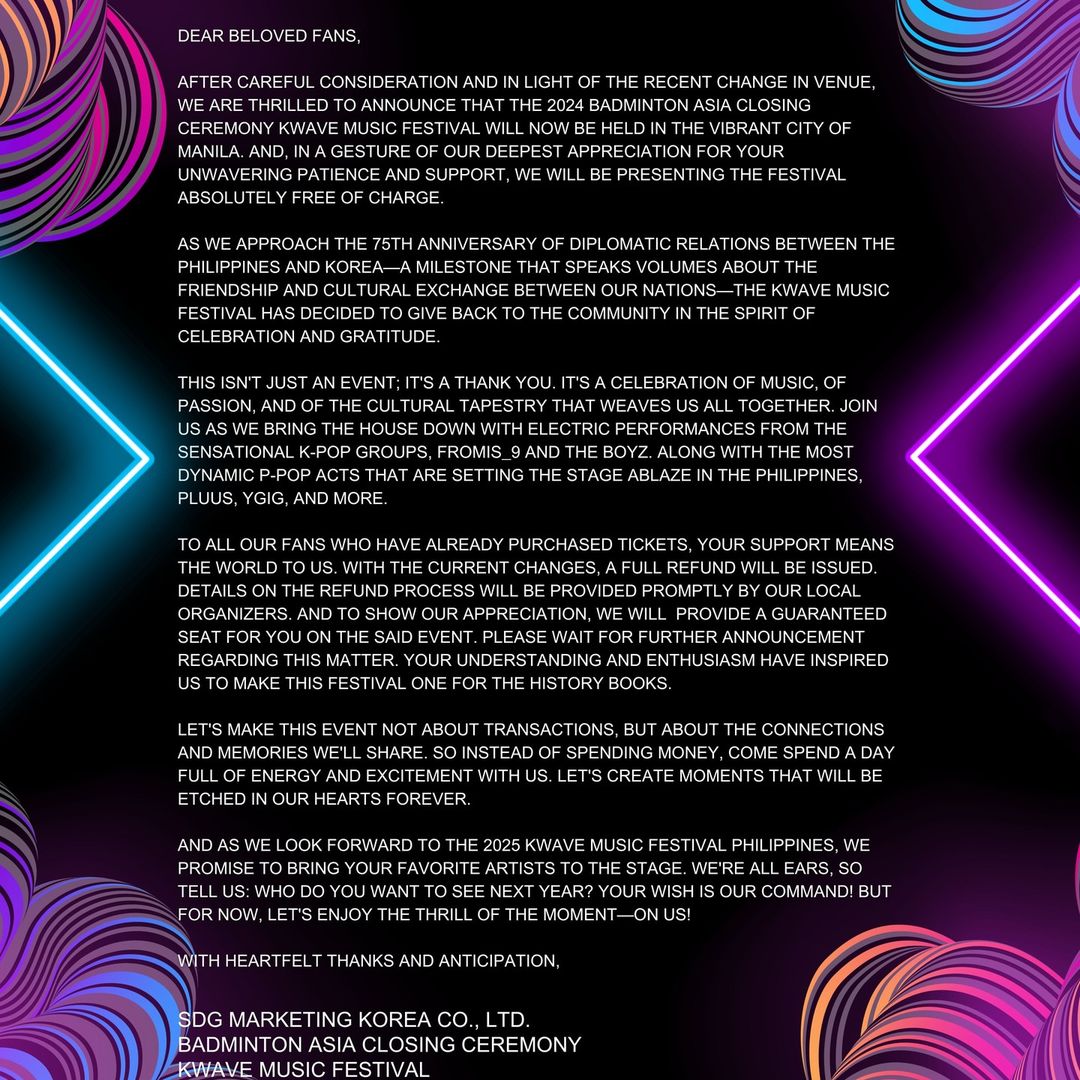The image is a large square with a solid black background. At each of the four corners, there are vibrant, neon-like swirling patterns. The upper left and lower right corners feature swirls in hues of purple, pink, gray, and black, while the upper right and lower left corners showcase blue, purple, and black swirls.

In the center of the image, occupying a left-aligned column of text, is an announcement written in all-caps white letters. The largest text at the top reads "Dear Beloved Fans." The first paragraph of the text explains: "After careful consideration and in light of the recent change in venue, we are thrilled to announce that the 2024 Badminton Asia Closing Ceremony K-Wave Music Festival will now be held in the vibrant city of Manila. In a gesture of our deepest appreciation for your unwavering patience and support, we will be presenting the festival absolutely free of charge." 

Following this introductory paragraph are several more paragraphs of similar content. The announcement concludes with, "With heartfelt thanks and anticipation," followed by the names "SDG Marketing Korea Company Limited" and "Badminton Asia Closing Ceremony K-Wave Music Festival." The neon colors and patterns add a festive and luminous touch to the announcement, emphasizing the celebratory nature of the event.